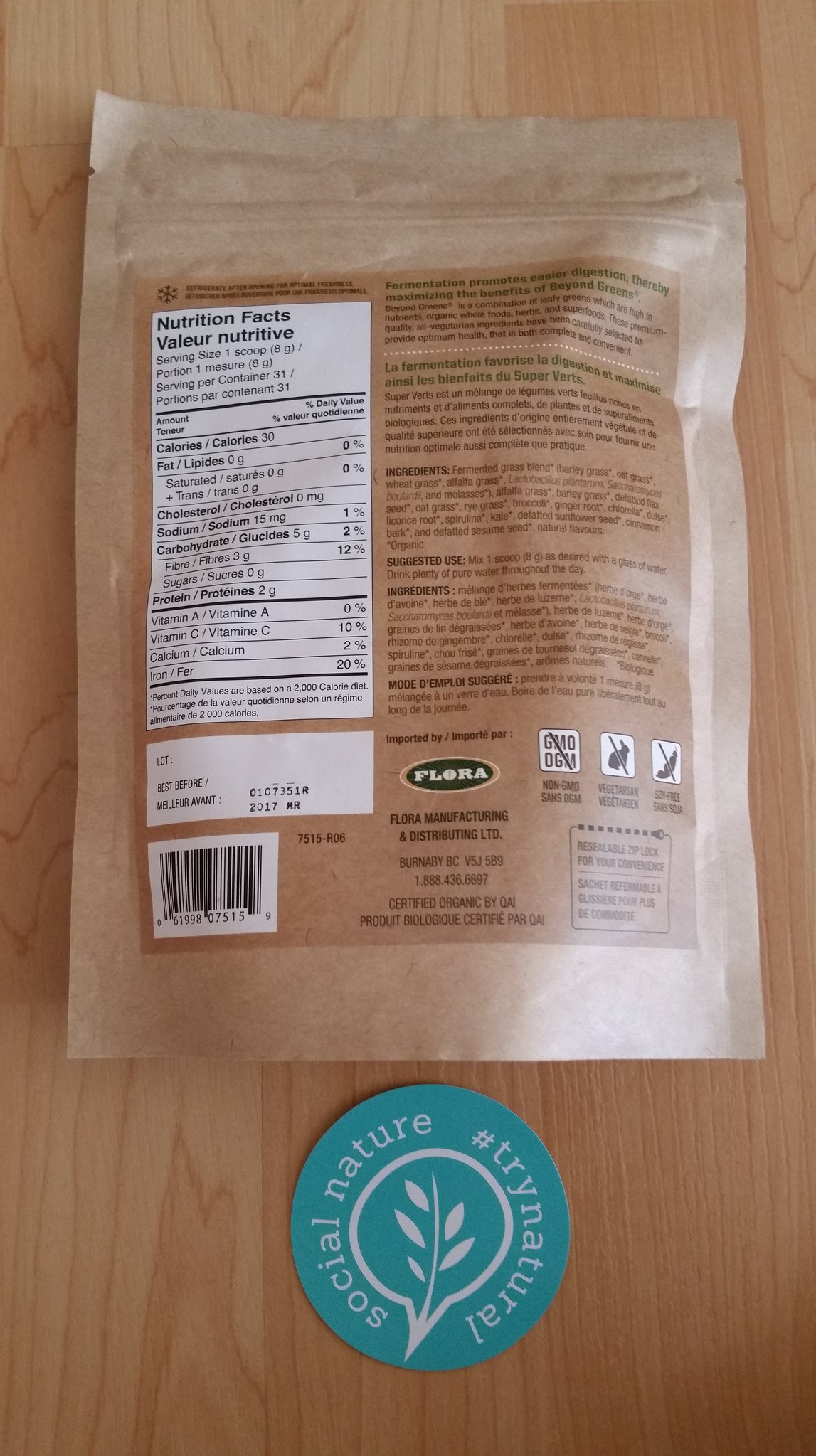This photograph features a food package and a sticker displayed on a light brown wooden tabletop. The tabletop features vertically running light-colored wood grain. The package is a plastic, envelope-style bag with a light brown hue, reminiscent of a brown paper bag. It includes a zipper at the top and a "tear here" notch for easy opening. The back of the package hosts a slightly darker brown rectangular label. This label is divided into sections: a white and black nutrition facts column on the left, detailed ingredients and company information in paragraph form on the right, and a barcode in the lower-left corner. Resting beneath the package is a light blue circular sticker featuring a white outline of a leaf in the center, bordered by the words "Social Nature" and "#TryNatural."